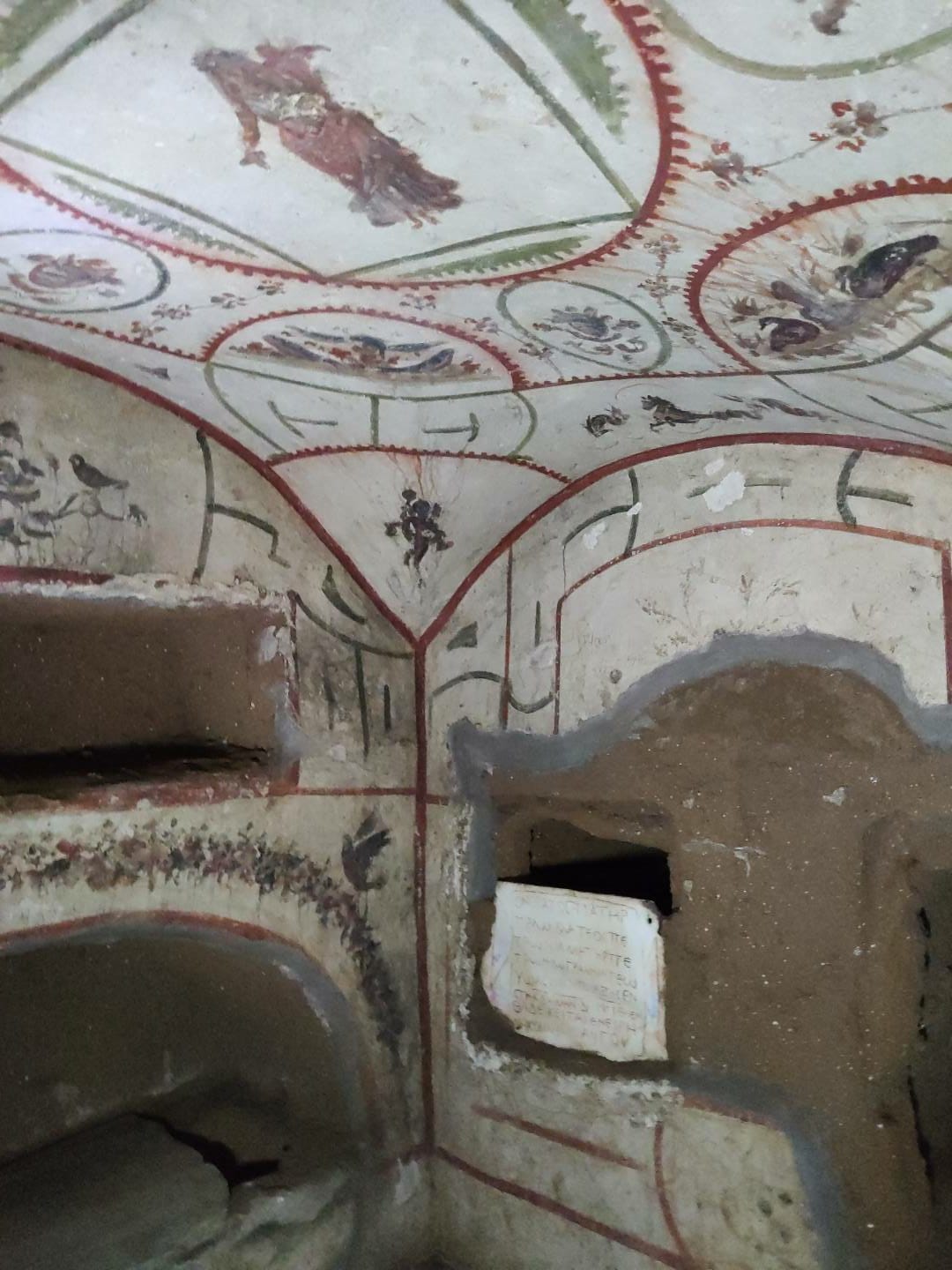The image depicts the interior of a highly weathered and aged room, potentially a bathroom, with walls and ceilings evocative of ancient cave art or tribal decor. The curved ceiling features a bold design reminiscent of a red cog wheel, complemented by green markings. The room's walls, which appear quite old and possibly unstable, exhibit a large brown panel surrounded by gray paint with a conspicuous hole. Built into the wall are several intentional cutout shelves and nooks, one of which holds a hanging towel. Decoratively aligned with the ceiling’s style and colors, the walls also house an image of a woman that looks Indian or tribal. The condition of the space suggests it has not been maintained for years, adding to its rustic and mysterious charm.